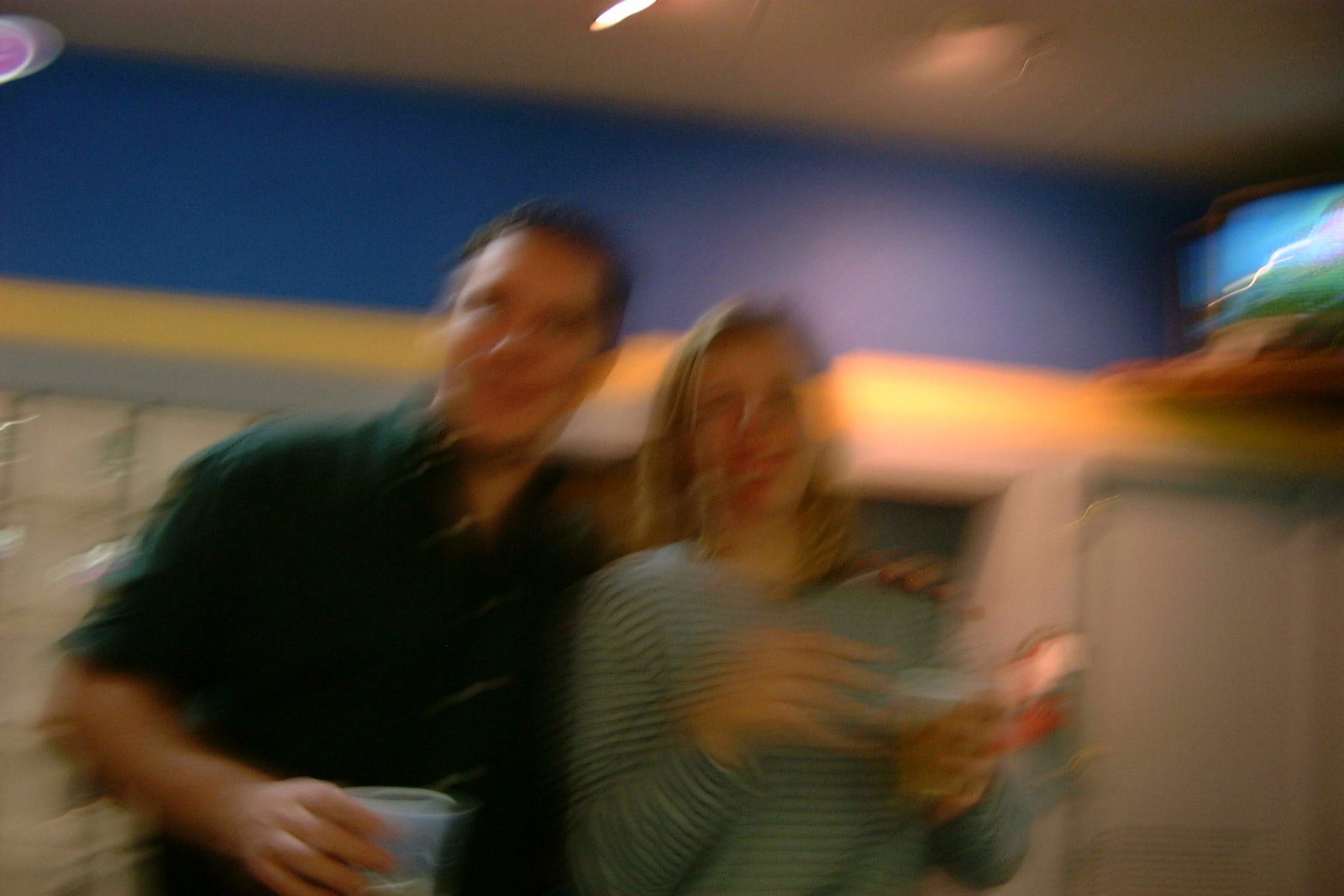In this extremely blurry photograph, a man and a woman stand closely together, facing the camera and appearing to smile. The man, positioned on the left, has short brown hair and a light skin tone. He is dressed in a green short-sleeved collared shirt with the sleeves rolled up. In one hand, he holds a plastic cup, while his other arm is affectionately around the woman's shoulder. The woman, beside him, has short blonde hair and is wearing a long-sleeved, blue collared shirt. She too is holding a plastic cup with both hands; one hand touches the side of the cup, containing what appears to be a yellowy-brown liquid. The background features a tri-colored wall: blue on the upper part, a yellow-orange stripe running horizontally, and white on the bottom. Additionally, a TV screen can be observed in the blurred upper right corner. The setting's ceiling is grey with visible lights. Despite the blurriness, the joyful expressions of the individuals are perceptible.